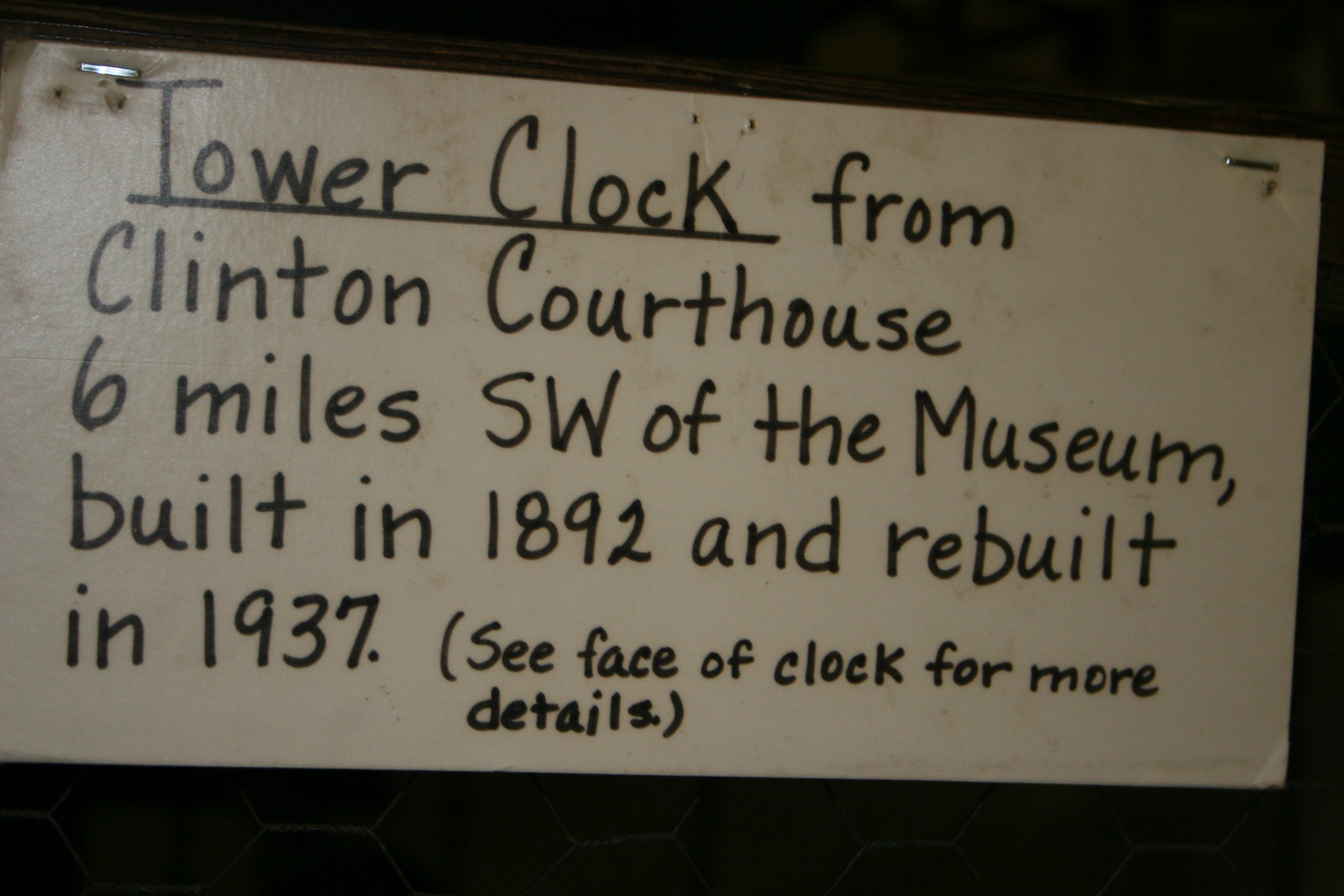This photograph depicts a worn, rectangular white piece of paper, slightly discolored and stained, attached to a background surface, possibly wooden, with two metallic pins or staples at the top left and top right corners. The paper features handwriting in black ink or marker, which reads: "Tower Clock" with both words underlined. Below this, more text follows: "From Clinton Courthouse, six miles southwest of the museum. Built in 1892 and rebuilt in 1937. (See face of clock for more details)." The paper looks older and the setting appears to be indoors, with dim lighting adding to the aged appearance of the document.